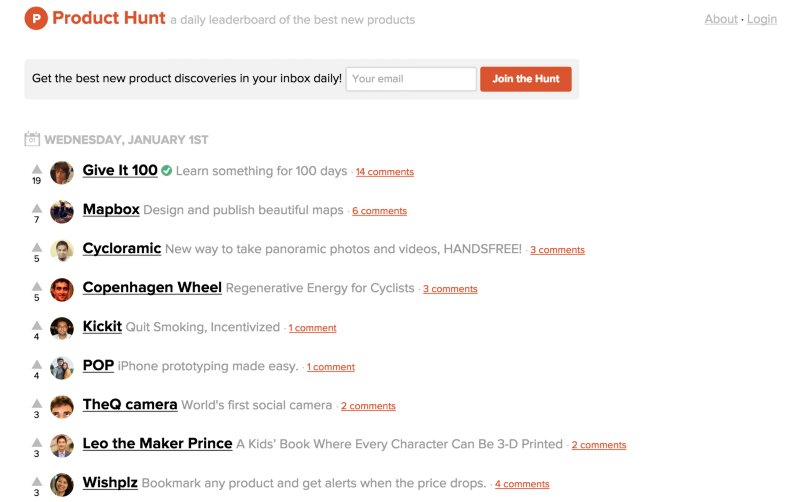The header displays the "Product Hut" logo on the top left, featuring a white 'P' set within an orange circle, with the text "Product Hut" in orange. Adjacent to this in gray text is the tagline, "A daily leaderboard of the best new products." On the top right, there are gray, underlined links for "About" and "Login."

Beneath the header, a gray band features a black text prompt: "Get the best new product discoveries in your inbox daily." Following this, there is an email input box accompanied by an orange button labeled "Join the Hunt" with white text.

Directly below, aligned to the left, the date "Wednesday, January 1st" is written in gray. A numbered list of nine items follows, each entry showcasing a product along with its description and the number of comments it has received:

1. **Give it 100** - Top one. Learn something for 100 days. (14 comments)
2. **Mapbox** - Design and publish beautiful maps. (6 comments)
3. **Panoramic** - A new way to take panoramic photos and videos, hands-free. (3 comments)
4. **Copenhagen Wheel** - Regenerative energy for cyclists. (3 comments)
5. **Kick it** - Quit smoking and scent advice. (1 comment)
6. **Pop** - iPhone prototyping made easy. (1 comment)
7. **The Cube Camera** - World's first social camera. (2 comments)
8. **Leo the Maker** - Prints kids' books where everyone's character can be 3D printed. (Number of comments not provided)